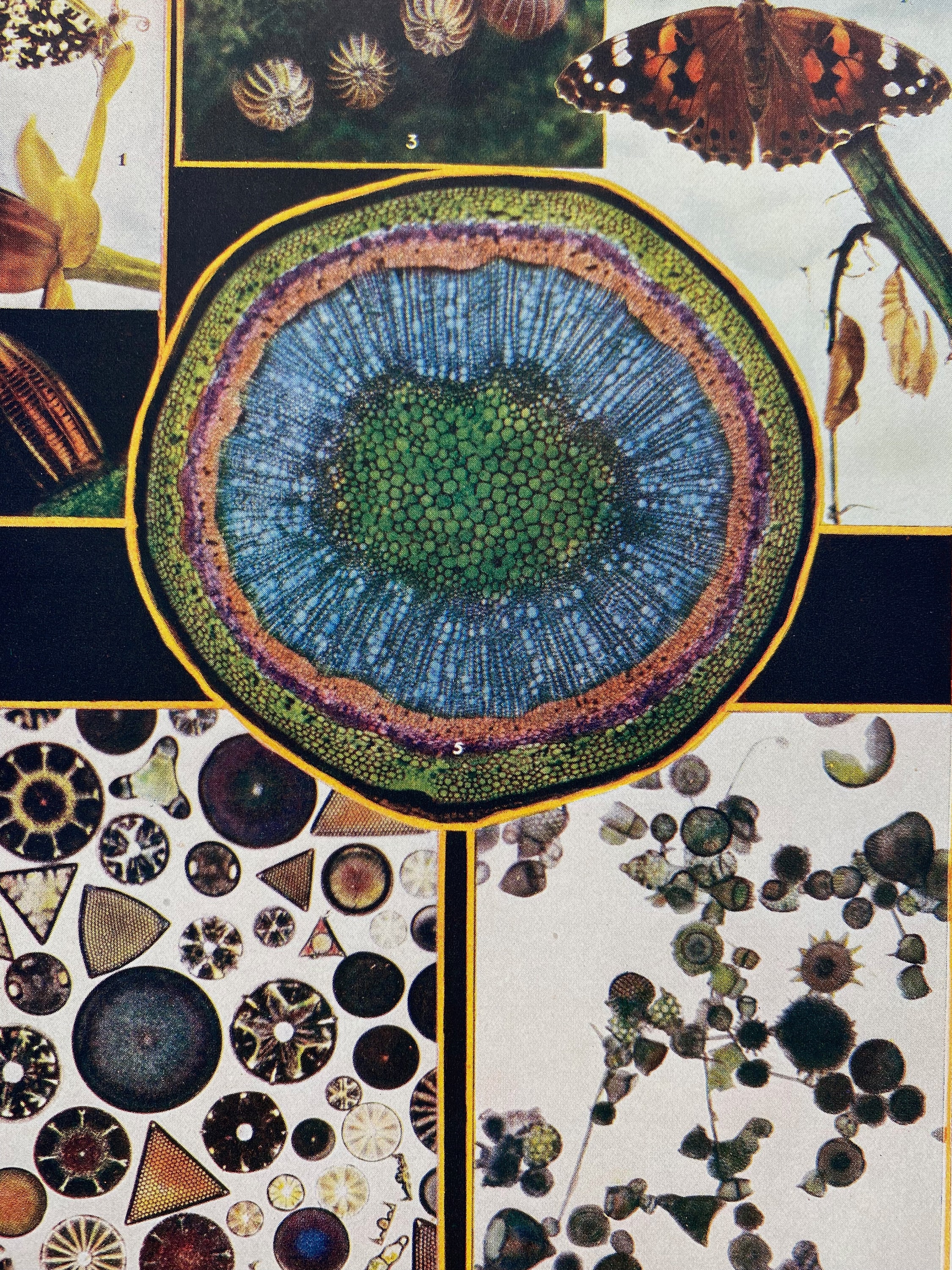The image is a collage of several pictures, each set in a distinct panel. In the top left corner, there’s the edge of a picture that goes off the image at the top and left. Next to it is a top panel featuring four spherical objects and the number three at the bottom. Just beneath it, a picture displaying a butterfly with orange, brown, black, and white wings perched on a branch extends off to the right.

Dominating the center and stretching from the top to the middle-bottom of the image is a large circular picture, which features multiple concentric borders. This circle has an outer yellow outline, followed by a black border, a green one adorned with dots, a thin purple border, a slightly thicker pink border, and, finally, a wide blue border. Within the innermost area, a cluster of small green circles forms the core.

In the bottom left corner, a panel showcases an assortment of objects of various shapes, including black circular objects, brown and light brown triangles, circular objects with a yellow star at the center, and another circle with a dark blue middle. Adjacent to it, on the bottom right, is an intricate picture of interconnected objects. These resemble flowers in black, brown, gray, and white hues connected by faint lines, or stems.

The upper left panel (partly off the image) resembles sea urchins against a green background, while the center displays another large circle with a yellow border, green interior, purple section, orange layer, and a larger blue part. At its core are multi-colored pebbles arranged in diverse shapes.

The panels are outlined by yellow borders with black negative spaces in between, adding structure to the vibrant assembly. Several images bear numbers — one in the top left panel, three in the top-right panel, and five in the central circular image. The collection also includes a variety of natural elements such as pebbles, flowers, butterflies, and sea urchins, each contributing to the multi-textured and colorful composition.